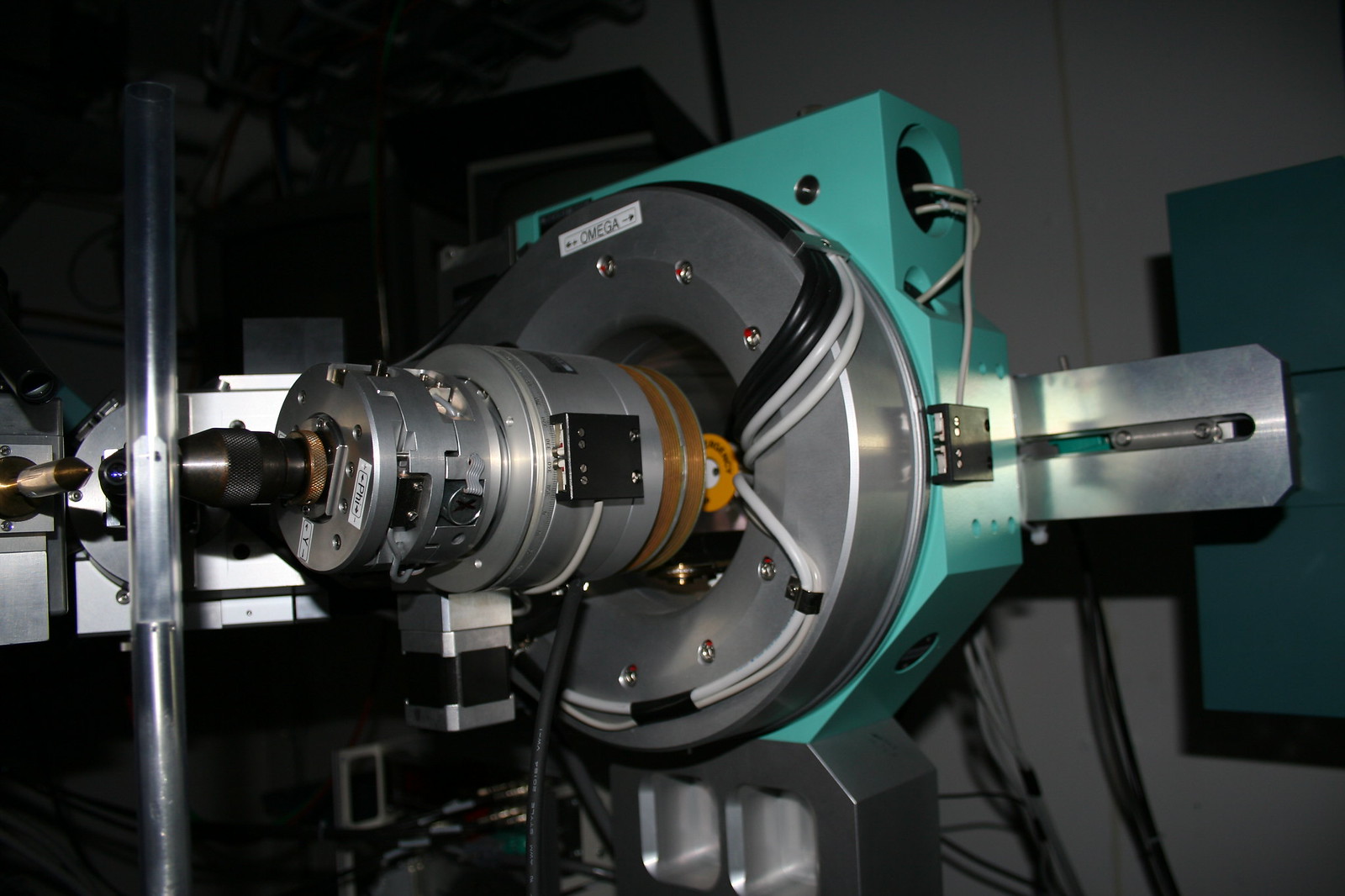This photograph, taken indoors in a dimly lit room, features a large, well-engineered piece of machinery that resembles industrial equipment more than a medical device. The primary structure of the machine is largely metallic gray with distinct aqua blue trim elements. The centerpiece is a prominent round metal component that suggests rotational functionality, reminiscent of a lathe. Additionally, two bullet-shaped protrusions flank the machine, with multiple wires extending from them and sprawling throughout the device and the room. Various smaller pieces of machinery and numerous wires populate the surrounding area, contributing to the impression that the setting might be a laboratory or an advanced manufacturing facility.